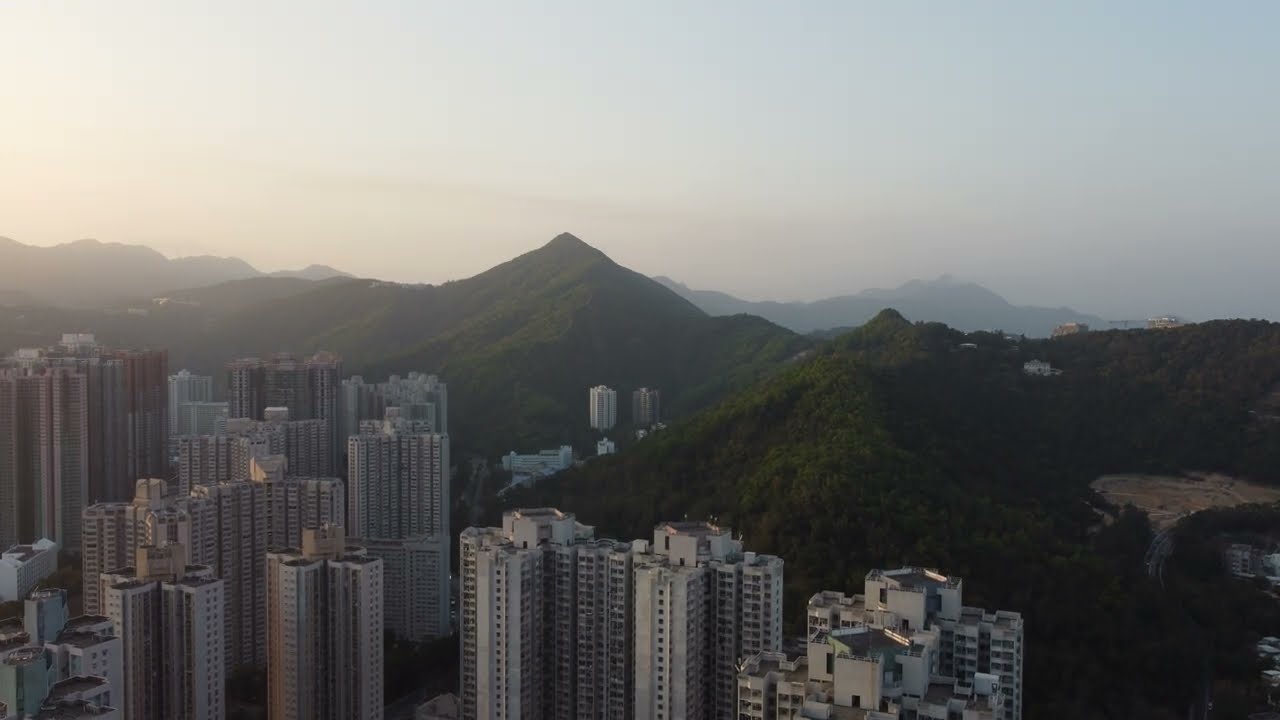This photograph captures a striking scene of a tropical island that has been heavily urbanized, showcasing numerous tall buildings that could be apartments or hotels. It's reminiscent of iconic cityscapes like Hong Kong but may also resemble places such as Oahu. The city area is densely packed with many high-rise buildings, some exceeding 10 stories, characterized by a modern, sterile appearance with numerous windows. Symmetry is evident in the design of the buildings, and one prominent structure features a part jutting out from the front, giving the impression of being split but connected.

To the right of the urban area, lush green tree-covered mountains rise dramatically, creating a stark juxtaposition between the bustling city and the serene, natural landscape. This surreal blend of urban and rural elements makes the scene particularly captivating. The photograph is set during dusk, with a slight orange hue illuminating the clear sky. Despite the overall clear sky, there is a hint of fogginess further up, adding to the unique atmosphere of the image. The mountains, valleys, and peaks form a picturesque backdrop that seamlessly integrates with the city below.